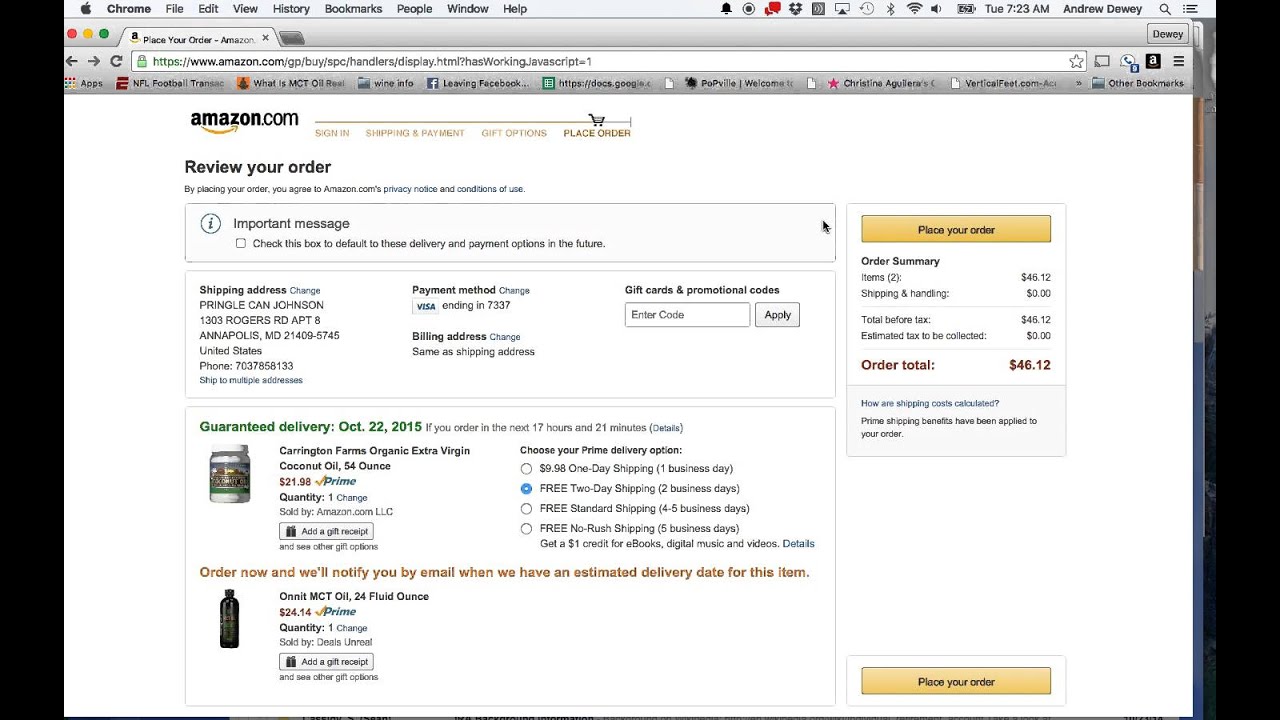This screenshot captures an Amazon ordering page on a Chrome browser on a Mac. At the top of the screen, the Apple logo is displayed, followed by menu tabs: Chrome, File, Edit, View, History, Bookmarks, People, Window, and Help. The top right corner indicates it is Tuesday at 7:23 AM, and the user logged in is Andrew Dewey.

The active Chrome tab is titled "Place Your Order - Amazon" with the address bar displaying Amazon's URL. The webpage prominently features a "Review Your Order" section under the "Place Order" tab with a shopping cart icon. 

Key details include an important message prompting users to default these delivery and payment options for future orders. The shipping address is listed as Pringle Can Johnson at 1303 Rogers Road, Apartment 8, Annapolis, Maryland, 21409, United States. The payment method is a Visa card, with the billing address identical to the shipping address. There is also an option to enter gift cards and promotional codes.

The order summary is detailed below:

1. Carrington Farms Organic Extra Virgin Coconut Oil, 54 ounces, priced at $21.98, with a guaranteed delivery date of October 22, 2015. The order quantity is one, and it qualifies for free two-day shipping.
2. Onnit MCT Oil, 24 fluid ounces, priced at $24.14. The notice states, "Order Now and will notify you by email when we have an estimated delivery date for this item."

The total order summary on the right side of the screen shows a total cost of $46.12 for the two items, with no additional tax applied. The "Place Your Order" button is highlighted in a yellow bar at the bottom right corner of the page, ready for the user to confirm the purchase.